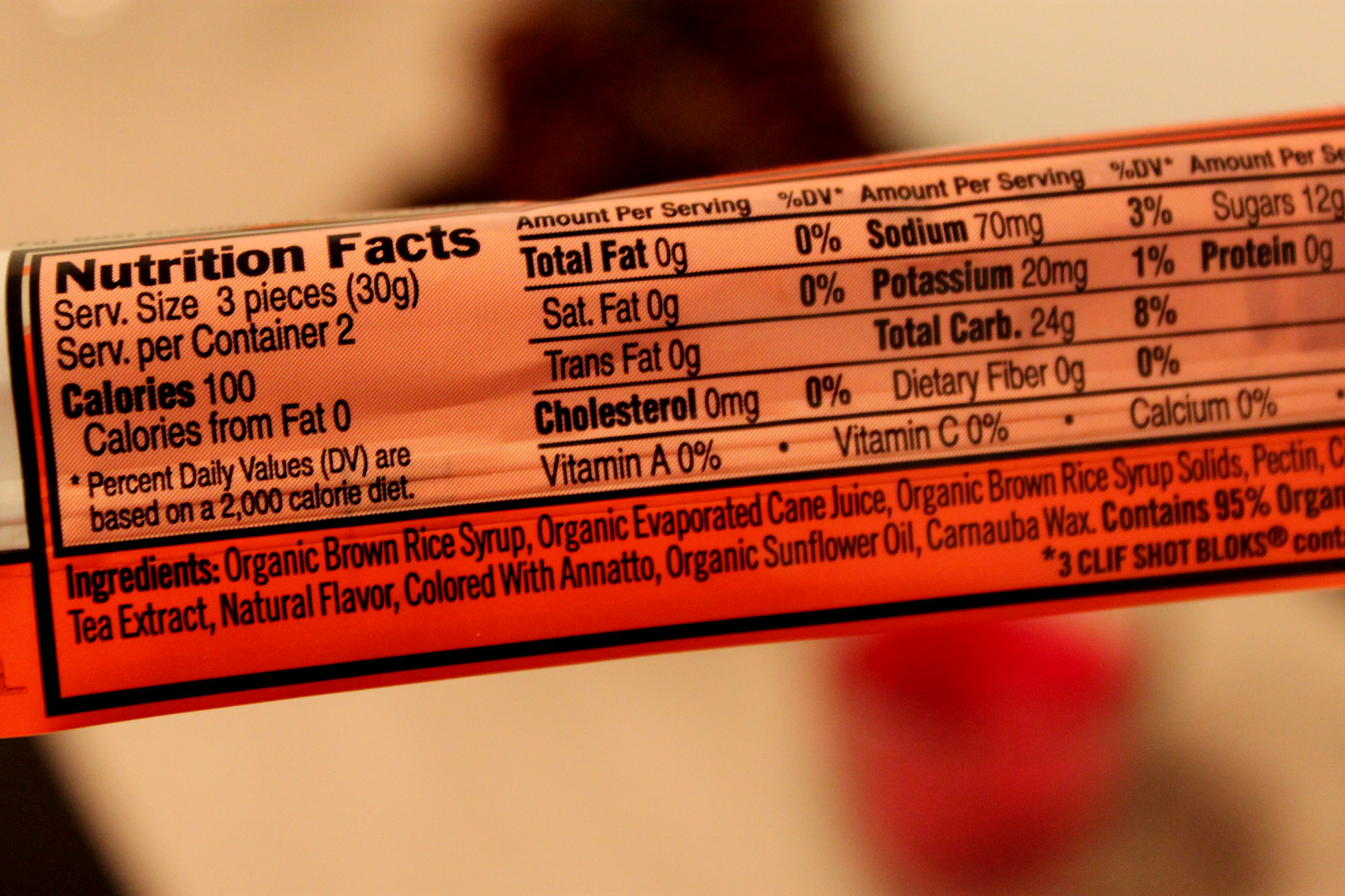This is a close-up image of a nutrition label that appears to be from a snack, possibly some kind of candy or energy blocks, specifically Cliff Shot Blocks. The label shows detailed nutritional information and has a serving size of 3 pieces (30 grams) with 2 servings per container. Each serving contains 100 calories, with 0 calories from fat. The amounts per serving and their respective percent daily values are as follows: Total fat, 0 grams (0%); Saturated fat, 0 grams (0%); Trans fat, 0 grams; Cholesterol, 0 milligrams (0%); Sodium, 70 milligrams (3%); Potassium, 20 milligrams (1%); Total carbohydrates, 24 grams (8%); Dietary fiber, 0 grams (0%); Sugars, 12 grams; and Protein, 0 grams. The ingredient list includes organic brown rice syrup, organic evaporated cane juice, organic brown rice syrup solids, pectin, tea extract, natural flavor, colored with annatto, organic sunflower oil, and carnauba wax, with the product containing 85% organic ingredients. The background of the image is out of focus, emphasizing the clear and readable details of the label.